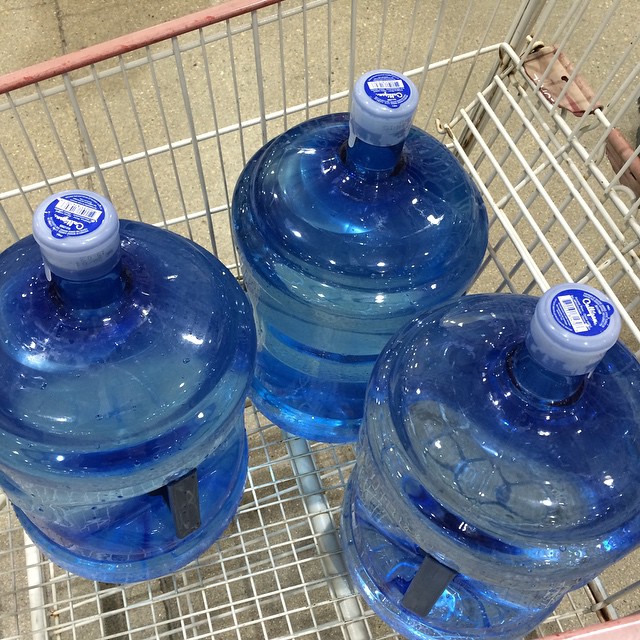In the image, a slightly worn and rusty shopping cart with white and chrome construction and red protective edging is seen on a gray, speckled laminate floor in a store. The cart carries three 5-gallon Culligan water bottles, made of clear blue-tinted plastic with black lifting handles. Each bottle is topped with a white cap featuring a blue circular insert marked with the Culligan logo, surrounded by small, unreadable text and a barcode. The cart's age and use are evident from its condition, and the lighting from above reflects off the water bottles, highlighting their glossy surface. The floor beneath the cart shows a mix of white, black, and brownish tiles, adding to the scene's detailed texture.